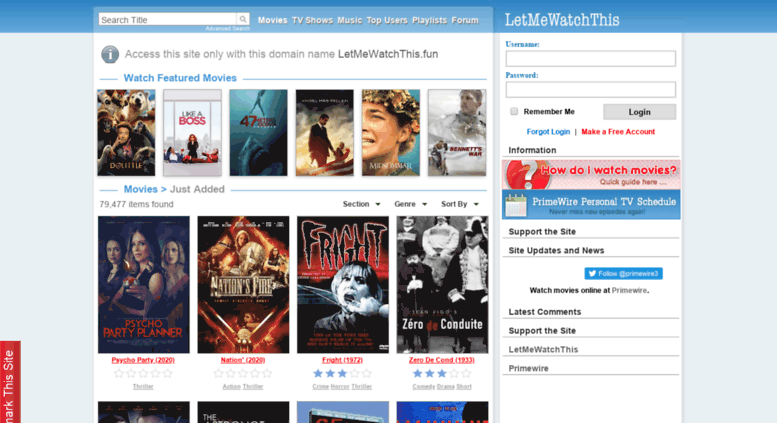This image is a screenshot from a web page, likely titled "Let Me Watch This," given the prominent display of this phrase in the header. The header itself is blue with white text on the right side spelling "LetMeWatchThis" as a single concatenated word using uppercase letters. To the left, the header contains a gray-colored font message that reads, "Access the site only with this domain name: letmewatchthis.fun."

Below the header, the page layout prominently features rows of movie posters, predominantly displaying horror films. Two full rows of posters are visible, along with the top edge of a third row at the bottom of the screen.

To the right of the movie posters, there is a vertical login form with spaces designated for a username and password. Just below the form, there is a small banner with a pink background and red text that asks, "How do I watch movies?" followed by a link titled "Quick guide here."

Further down, there is a section with a blue background and white text that reads "PrimeWise personal TV schedule." Under this section, there are several links including "Support this site," "Site updates and news," and "Latest comments." There is also repeated mention of "Support this site," "Let Me Watch This," and "PrimeWise," likely serving as hyperlink buttons for easy navigation around the site.